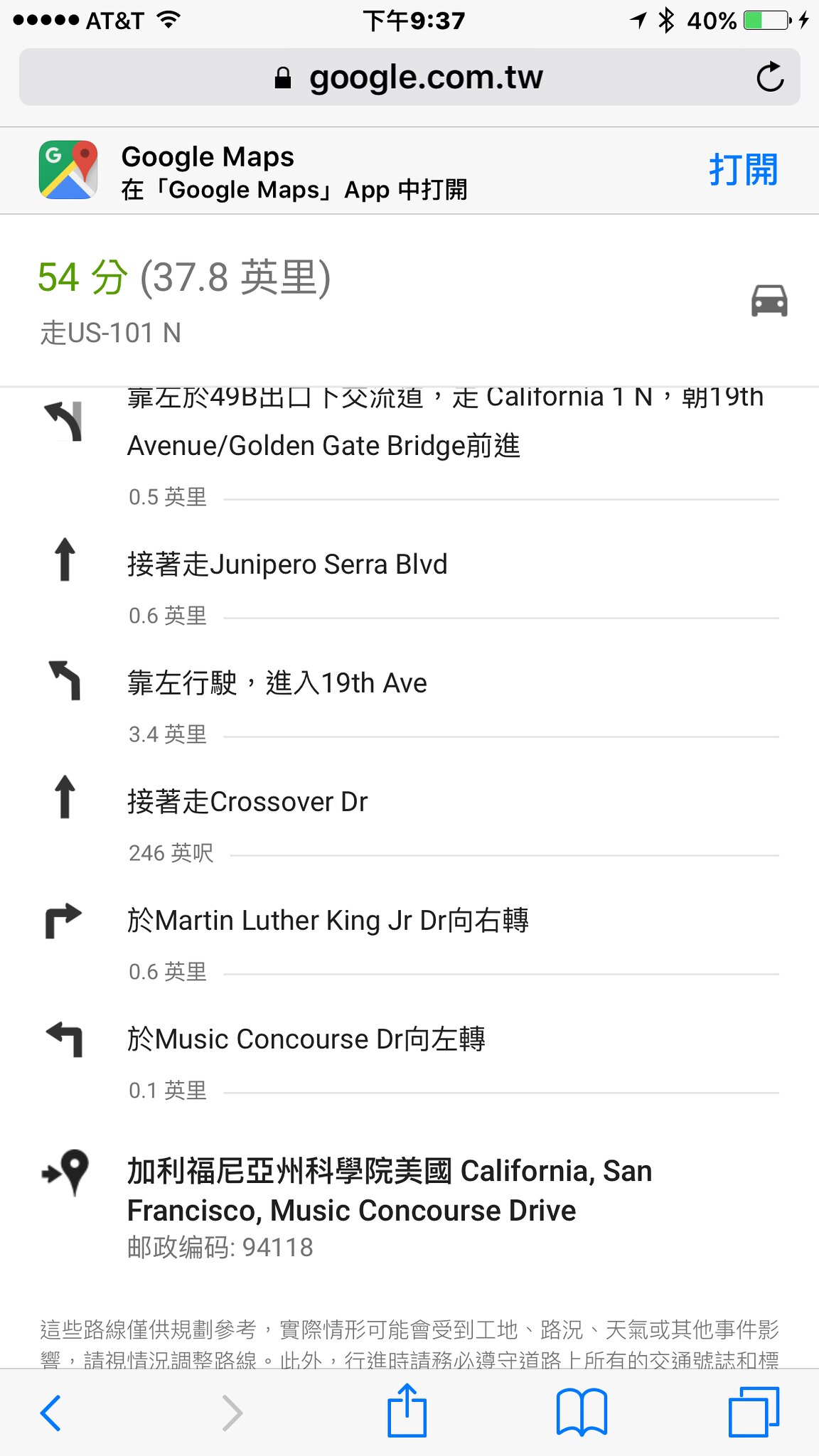This image is a detailed screenshot of Google Maps directions displayed in the Safari web browser on an iPhone, clearly identifiable by the distinct Safari interface. At the top of the screen, the address bar prominently shows "google.com.tw," indicating that this is the Taiwanese version of Google. The iPhone status bar includes recognizable icons such as the AT&T logo, Wi-Fi, Bluetooth symbols, and a battery meter, further confirming the device type. Below the address bar, a light gray rectangular section displays the Google Maps logo followed by "Google Maps" and subsequent Chinese characters. The directions are listed on a white background, with turns indicated by arrows aligned to the left. Each instruction includes Chinese characters followed by their English translations. Notable elements include a green number 54 and a "37.8" in parentheses accompanied by Chinese text, possibly indicating distances or specific route markers. The detailed format and bilingual text are typical of Google Maps' navigation interface.